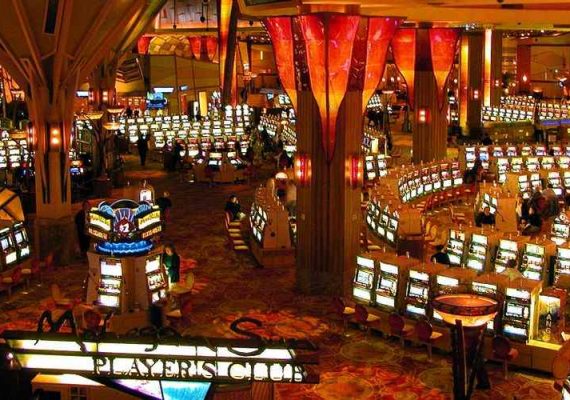This indoor photograph captures the vibrant and lively atmosphere of a casino, dominated by a vast array of slot machines. The machines are arranged in both traditional rows and in more unique, circular formations where players can sit around and face one another. The scene is illuminated by the bright lights of the slots, which contrast strikingly with the predominantly dark brown and orange carpeting.

The image, taken from an elevated perspective, reveals rows upon rows of slot machines stretching into the distance, all switched on and showcasing their white lights. Centrally located pillars, adorned with long, bright red lights extending to the ceiling, contribute to the casino's dramatic ambiance.

Towards the bottom left of the image, a sign reading something akin to "Megan's Players Club" hints at a dedicated area for club members. The overall palette of the photograph includes hues of orange, red, brown, blue, and purple, creating a warm but somewhat subdued lighting environment. This detailed depiction emphasizes the overwhelming presence of slot machines, underscoring the casino's intense, activity-filled atmosphere.